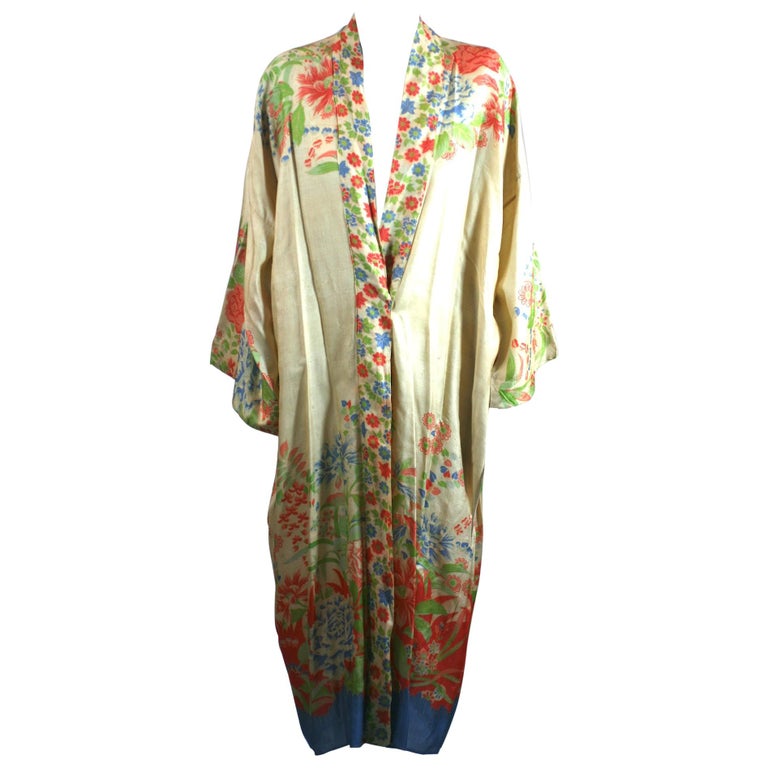The photograph showcases a traditional, long female dress, reminiscent of a kurta or robe, set against a white background. The predominantly cream-colored garment features an extensive array of floral and leaf designs in red, green, and blue hues. These intricate patterns adorn several areas of the dress, including the neckline, shoulders, wrists, and borders, extending to a heavily decorated bottom hemline. The dress, which appears to have a V-neck and loose, frilly long sleeves, also exhibits a distinctive band adorned with floral motifs that starts at the shoulders, meets at the abdomen, and continues down to the hem. The lower portion of the dress transitions into a blue stripe at the bottom, contributing to its elaborate and traditional aesthetic.